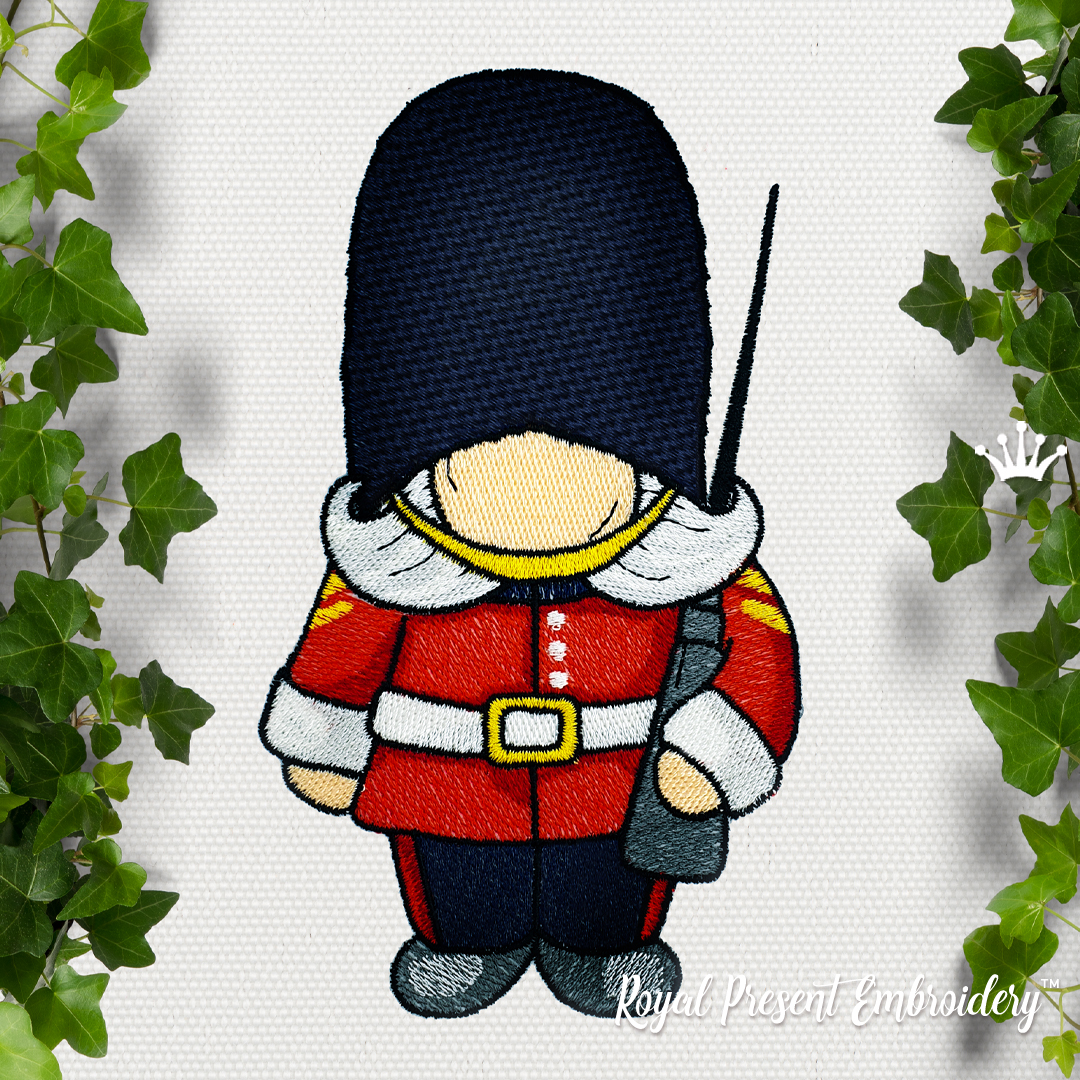The image is a detailed photograph of an intricately embroidered British royal guard, sewn onto a thick, white fabric. The central figure is a British soldier, identifiable by his red and white jacket, blue slacks with red stripes on either side, and black shoes. He carries a rifle slung over his shoulder and sports a tall, black, bear-skin hat, approximately three inches tall, with a gold strap under the chin. Notably, the soldier's face is a blank white oval without any features, and his hands are simple ovals with no fingers. Flanking the soldier are long pieces of green ivy, adding a decorative touch. On the right side of the image is a crown, and the bottom right corner features the cursive text "ROYAL PRESENT EMBROIDERY" with a small "TM" denoting it as trademarked. The meticulous detail and composition suggest a high-quality piece of embroidery, possibly signifying a royal association with its regal imagery and text.